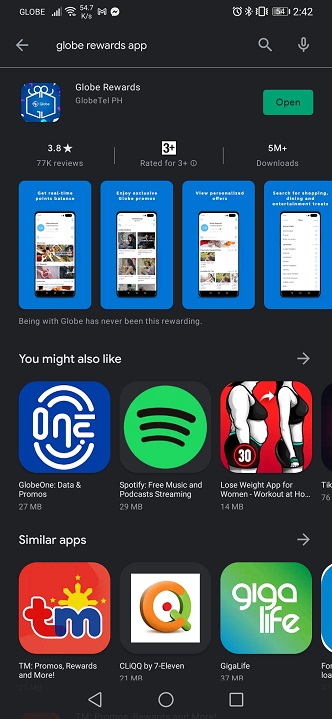In this screenshot of the Google Play Store app page for the Globe Rewards app by GlobalTellPH, the user has searched for "Globe Rewards app," as indicated in the search bar at the top of the screen. The status bar above the search bar displays the current time (2:42 PM), a fully charged battery (100%), and full network signal strength with Globe as the carrier.

The main section of the page highlights the "Globe Rewards" app, which has garnered a rating of 3.8 stars based on 77,000 reviews. It is suitable for users aged 3 and up and has achieved over 5 million downloads. The app's promotional tagline, "Being with Globe has never been this rewarding," suggests a focus on customer rewards and benefits.

Four informative screenshots of the app outline its key features: 
1. "Get exclusive perks and discounts"
2. "Enjoy exclusive Globe promos"
3. "View and redeem rewards"
4. "Earn rewards for your everyday activities"

Below the app's details, there is a section with similar or recommended apps, including "TM Promos and Rewards," "Click by 7-Eleven," and "Giga Life." This page comprehensively provides users with all essential information about the Globe Rewards app, from its functionalities and user ratings to other app suggestions.